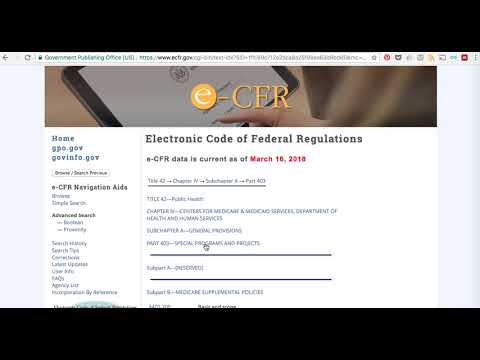The image features a government document interface framed by thick black bars at the top and bottom, as well as on the left and right sides. In the top black bar, green text reads "Government Publishing Office" followed by a URL beginning with "https." A red circle highlights a grey icon on the screen. Below this, a picture displays a tablet showing the words "e-CFR" (Electronic Code of Federal Regulations), suggesting someone is accessing regulatory information on the device.

Adjacent to this, the interface shows a navigational panel with links labeled "https.gov," "government.gov," "e-CFR," "Navigation Aids," and "Advanced Search." Text on the screen indicates the electronic data is current as of March 16. Specifically, Chapter 4 of the document is highlighted. There are grey bars flanking the left and right sides of the chapter text, which appears to detail part of the electronic code of federal regulations. The overall layout seems to be an official digital platform for accessing federal regulatory information.